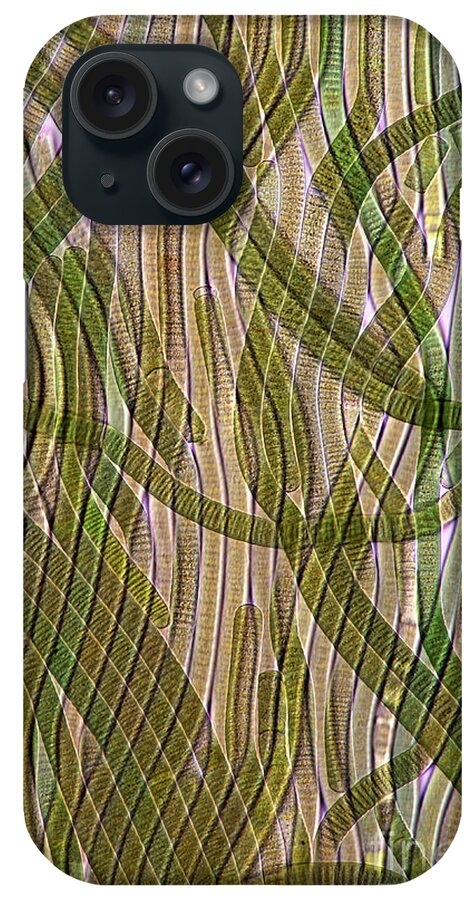The image showcases the back of an iPhone, likely a more affordable model, as it features two large cameras along with a smaller white dot and tiny gray dot. The phone is encased in a distinctive hardback phone case with rounded corners. The case exhibits a unique and irregular design characterized by thin, elongated lines that stretch from the top to the bottom. These lines, in muted hues of green and brown, serpentine randomly across the surface, evoking imagery akin to worms, microscopic creatures, or even ropes. The design is reminiscent of something one might see under a microscope, lending the case an intriguing, almost scientific appeal. There are no additional elements such as text or people in the image; the focus is solely on the phone and its captivating case.